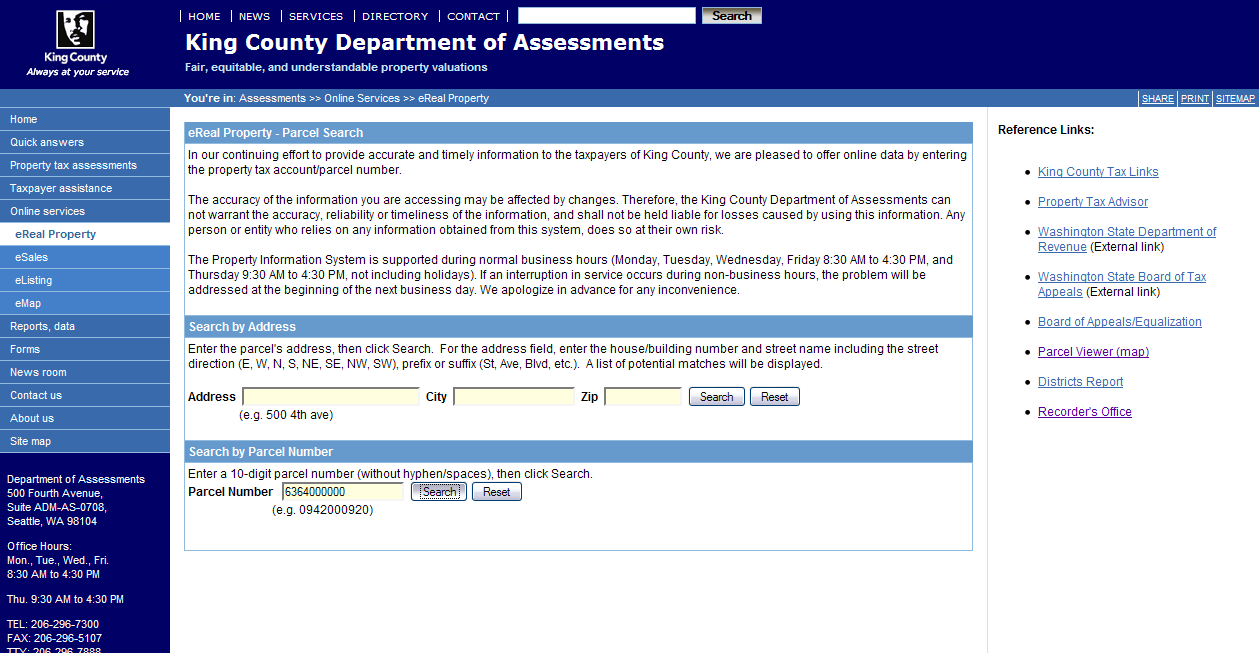Screenshot of King County Government Website – eReal Property Tab:

The screenshot captures the King County government website based in Seattle, Washington. The interface is structured with a dark blue navigation bar running horizontally across the top. The left sidebar, shaded light blue, features numerous navigation options: Home, Quick Answers, Property Tax Assessments, Taxpayer Assistance, Online Services, eReal Property, eSales, eListing, eMap, Report, Data, Forms, Newsroom, Contact Us, About Us, and Sitemap. Below these options, the contact information and business hours of the department are presented in dark blue.

Currently, the eReal Property tab is highlighted in the main display section featuring a white background. The tab focuses on the eReal Property parcel search. A text description informs users about the online data service, stipulating that while the King County government endeavors to provide precise and timely information, they cannot guarantee the accuracy, reliability, or timeliness of the data. Users are advised that reliance on the information is at their own risk and that any potential inaccuracies might arise from system updates or changes.

The website indicates that the property information system is maintained during normal business hours: Monday, Tuesday, Wednesday, and Friday from 8:30 AM to 4:30 PM, and Thursday from 9:30 AM to 4:30 PM, excluding holidays. In case of service interruptions during non-business hours, issues will be addressed at the next business day.

Two main sections for searching property information are available:

1. **Search by Address**: This section includes fields to input Address, City, and Zip code, accompanied by Search and Reset buttons.
2. **Search by Parcel Number**: This section instructs users to enter a 10-digit parcel number without hyphens or spaces into a search bar, followed by options to either Search or Reset.

The layout facilitates user navigation and access to property data, emphasizing both usability and transparency regarding the accuracy and limitations of the provided information.